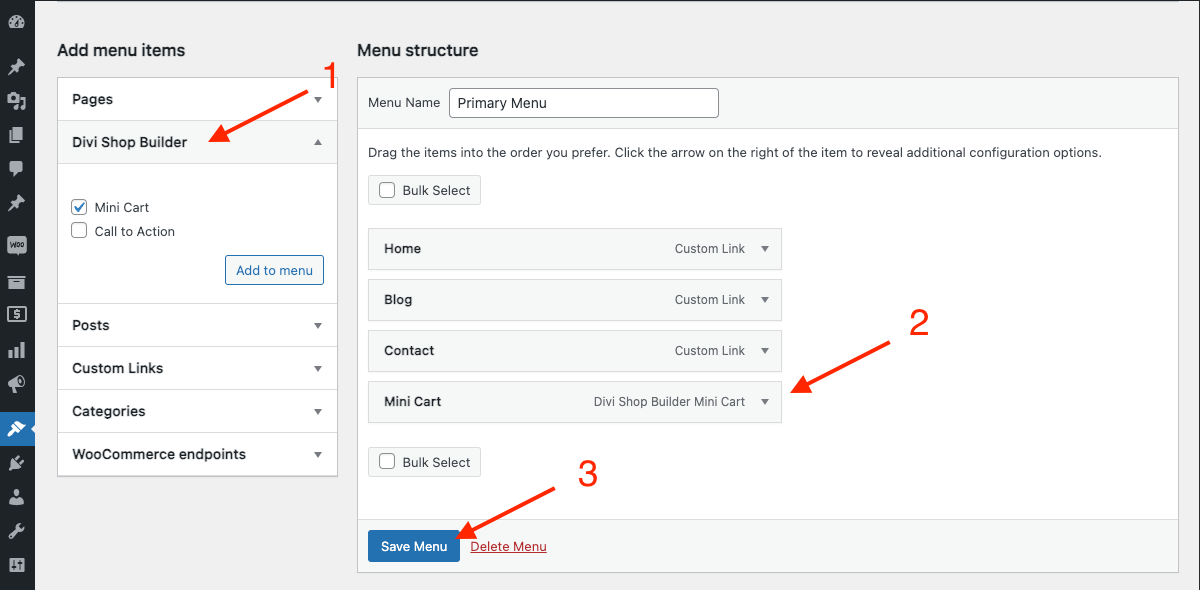The screenshot depicts a WordPress admin page with a focus on managing website menus. The interface features a very dark gray, narrow sidebar on the left, contrasting with the light gray background of the main page. Adjacent to this dark sidebar is a wider, white sidebar titled "Add Menu Items," which includes a list of items such as "Pages" and "DIBI Shop Builder," suggesting an integration with WooCommerce for e-commerce functionalities.

Highlighted within this sidebar, a red arrow labeled with the number "1" points to "DIBI Shop Builder," indicating its importance or relevance. The main content area of the page, situated to the right, includes various elements for menu configuration. Within this section, at the bottom-left corner, a blue rectangular button labeled "Save Menu" in white text is also marked by a red arrow with the number "3," signifying its crucial role in saving updates. Additionally, a gray rectangular drop-down menu, displaying "Mini Cart" on one side and "DIBI Shop Builder Mini Cart" on the other, is highlighted by a red arrow labeled "2," emphasizing its functional significance in the menu setup process.